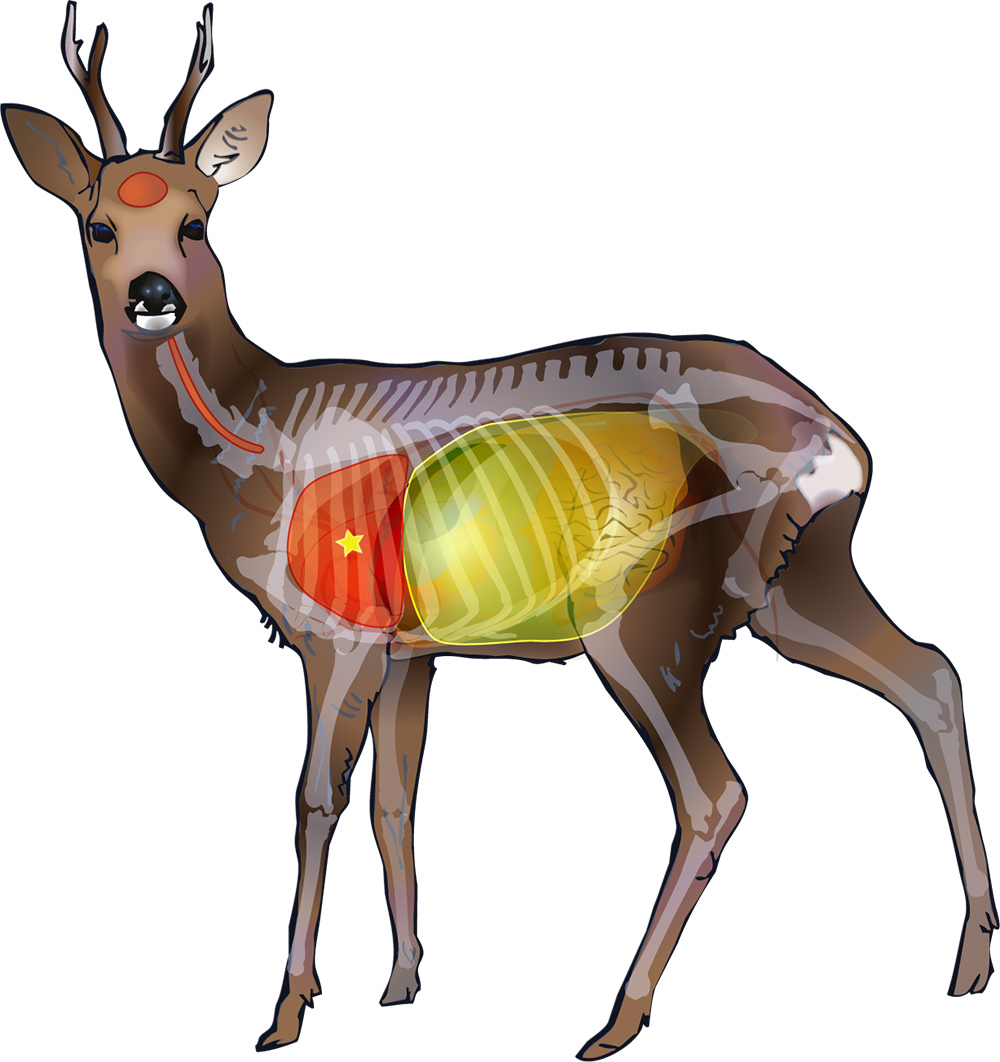This image is a detailed and unique computer graphic artwork of a deer, set against a stark white background. The deer, likely a male given its small antlers, has a transparency that allows viewers to see its internal anatomical structures. Prominently, a red circle adorns its forehead, leading down to its black eyes and nose. Through its translucent exterior, the deer’s vertebrae, spine, and ribcage can be clearly seen. The ribs arc down across the back, while the hip muscles and joints are visibly connected to the legs.

Notably, the depiction highlights various organs with distinct colors: a large red area, likely representing the heart, complete with a yellow star embedded in it, and an adjoining large yellow shape suggesting part of the stomach. The intestines also appear, coiled behind other organs. This artistic rendering gives a comprehensive view of the deer's internal anatomy in an infographic style, despite the absence of any text. The curious yellow star and red shapes, combined with the intricate depiction of bones and muscles, create a visually compelling and educational piece.